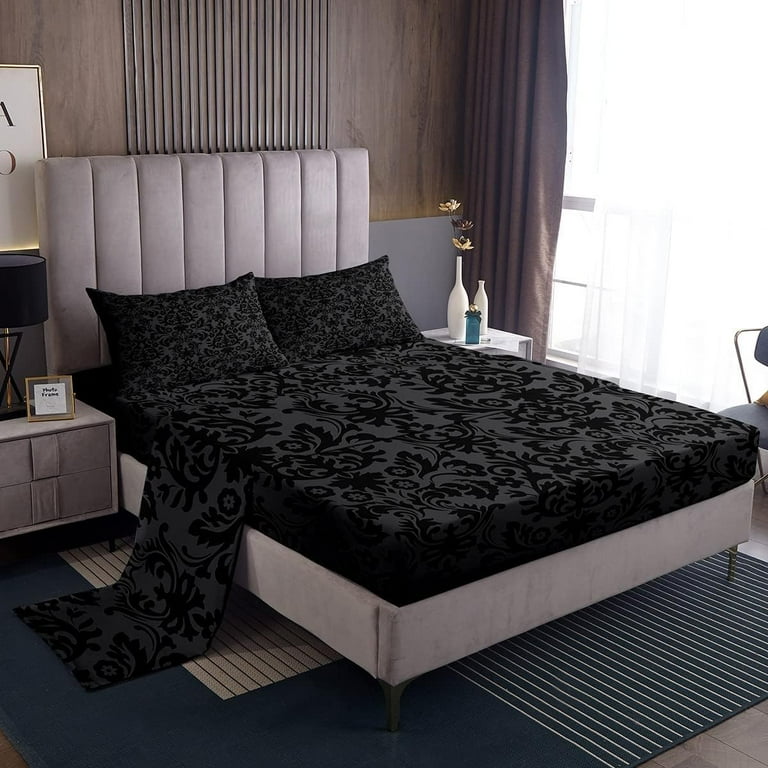This image depicts a well-appointed bedroom, featuring a plush bed with a large, quilted off-white headboard. The bed is dressed in black brocade sheets, with two matching black pillows, and a black sheet drapes over the left edge. The mattress base is a contrasting white. The room has a blue and white striped carpet with a darker blue central area.

The wall behind the bed is wooden with a textured finish, adding a rustic charm to the space. On the right side of the bed, there is a large window with brown curtains pulled to one side, allowing natural light to filter into the room. Below the window is a white nightstand, adorned with two white vases—one holding yellow flowers—and a smaller blue bottle with a gold cap.

On the left side, another nightstand stands, notable for its black lamp with a matching black shade. This nightstand also holds a gold-framed picture and a small note. The overall ambiance of the room combines cozy comfort with elegant details, creating a balanced and inviting environment.